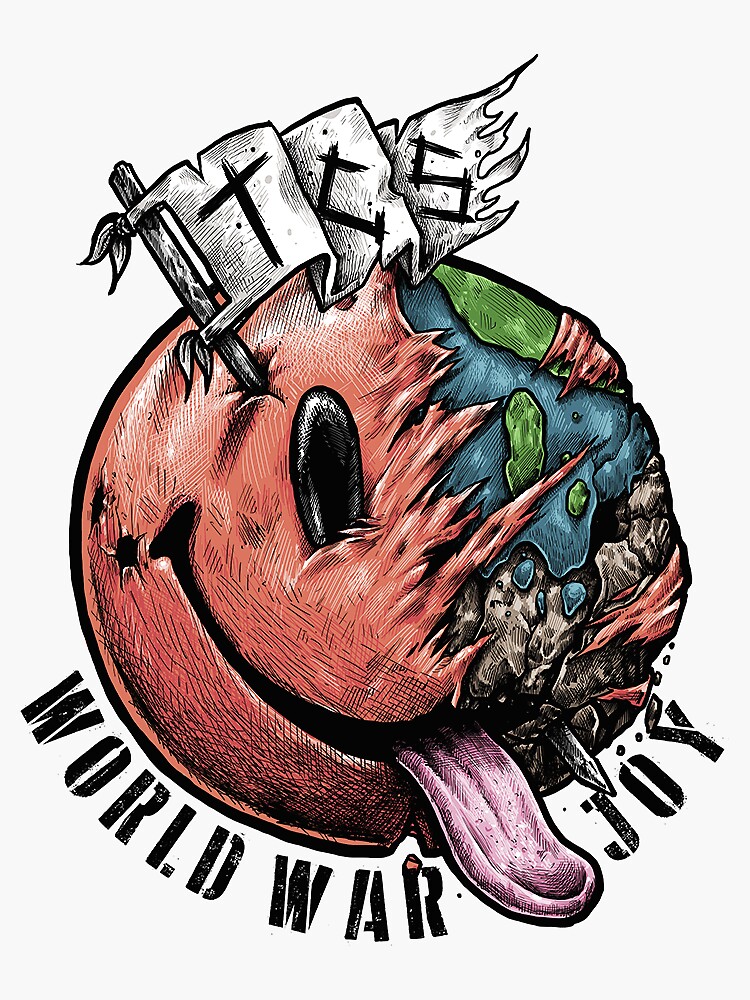This unique and detailed illustration, primarily a cartoon drawing, features a distinctive red smiley face with black crosshatching for shading. The face has a large black eye and a wide grin, with a pink tongue sticking out towards the lower right. The right side of the smiley face is partially stripped away, revealing an intricate landscape resembling a globe with white and green patches beneath the surface. 

A wooden spear pierces through the head, and at the top of this spear, a frayed banner with the letters "TCS" is attached. The left side of the face is significantly weathered, showing more signs of wear and tear, and the overall expression suggests a blend of chaos and joy.

Below the pink tongue and along the bottom of the smiley face, the words "World War Joy" are prominently displayed, indicating the title of the Chainsmokers' World War Joy Tour. The entire image is set against a white background, enhancing the striking colors and details of the artwork.